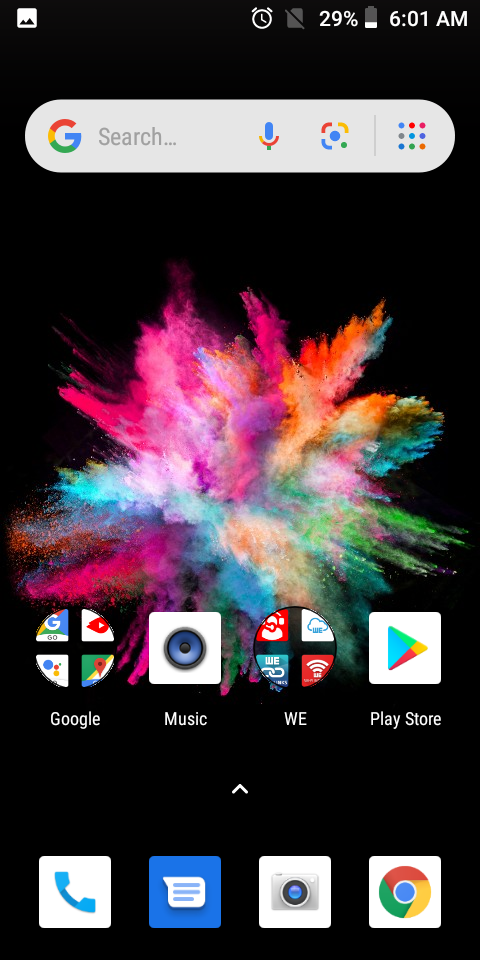This image is a screenshot of a smartphone displaying the home screen with a striking colorful graphic. The primary background is mostly black, which makes the vivid central graphic stand out—a dynamic explosion of colors resembling a dust cloud, featuring shades of white, blue, purple, magenta, orange, and green.

At the top left corner, there is an icon for a photo app. Moving towards the right, the status bar includes several icons: an alarm clock, a grayed-out square with a slash through it, indicating some form of deactivation, a battery icon showing 29% remaining charge, and the time, which is 6:01 a.m.

Below the status bar lies a light gray oval with a Google search bar. The search bar includes a capital "G" in Google's distinctive colors (red, yellow, green, and blue), the words "search..." in light gray, a microphone icon, a camera icon, and a grid of nine small dots arranged in a 3x3 fashion, also in Google colors.

At the bottom of the screen, there are eight app icons. The first is a folder containing several Google apps, followed by individual icons for a music app, an app with the initials "WE," and the Google Play Store. Centered at the bottom are icons for fundamental utilities: a phone, messaging, the camera, and Google Chrome.

This eye-catching and busy screenshot intricately displays the various elements and utilities present on the user's smartphone home screen, balanced against a vividly colorful background.